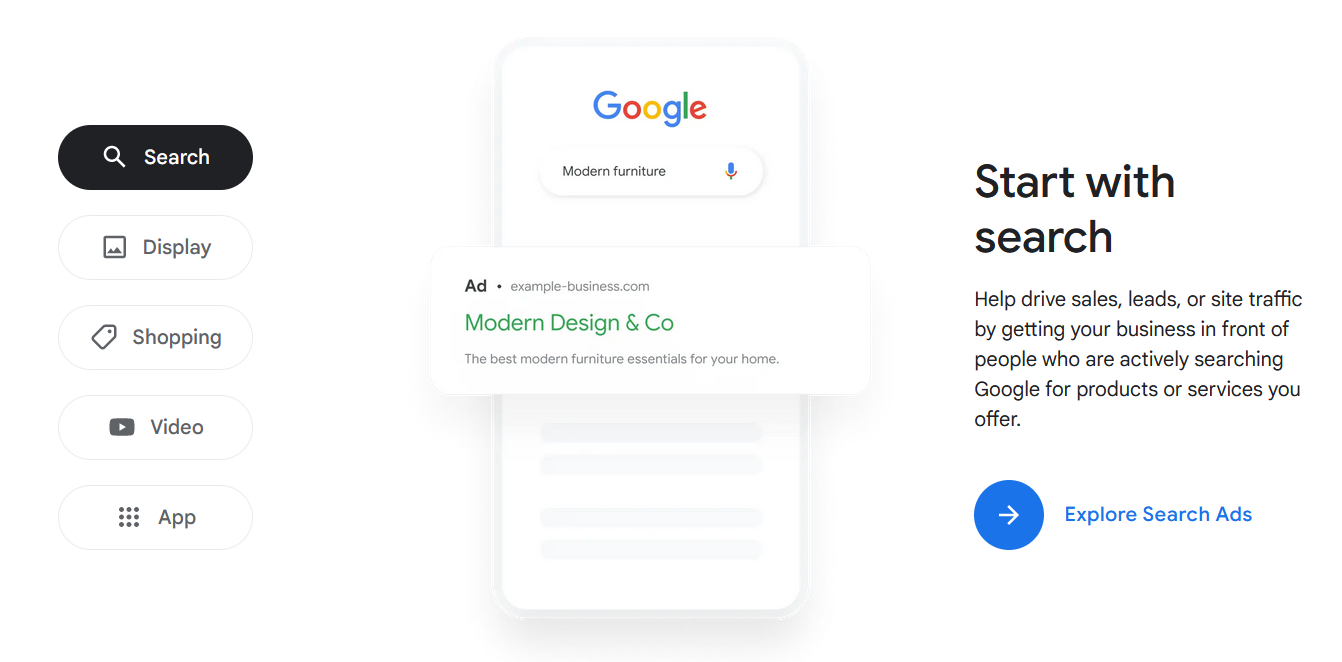Here is the detailed and cleaned-up caption for the described image:

---

This image appears to be a screengrab of a website interface. On the left side, there is a vertical navigation menu with several icons and labels. The first menu option is "Search," highlighted in black with white text, accompanied by a magnifying glass icon. "Search" is written with a capital 'S'. Below it is "Display," marked with a capital 'D' and an icon resembling a small mountain within a square. The next option is "Shopping," capitalized 'S,' featuring a price tag icon. Following that is "Video" with a capital 'V,' accompanied by a YouTube play button icon. The final menu option is "App," with a capital 'A,' depicted with a cluster of circles.

To the right of the menu, there is a simulated outline of a cellphone, shown in a whitish-grey hue. The screen displays the Google logo with letters in blue, red, gold, blue, green, and red, respectively. Below the logo, there is a search box. Inside the box, it reads "Modern Furniture" with a capital 'M' in "Modern." Adjacent to the search box is a red and blue microphone icon.

Below the search box, there is a black and green advertisement pop-up. It reads "ad examplebusiness.com, modern design and co. The best modern furniture essentials for your home." Further down, in black text, there is a message stating: "Start with search: help drive sales, leads, or site traffic by getting your business in front of people who are actively searching Google for products or services you offer."

At the bottom, a call-to-action states: "Explore Search Ads" with 'Explore' having a capital 'E', 'Search' a capital 'S', and 'Ads' a capital 'A', all highlighted in blue. Next to it is a blue circle with a white arrow. The text is of excellent quality, visually bold, and user-friendly for individuals with low vision.

Nothing else of note is present in the image.